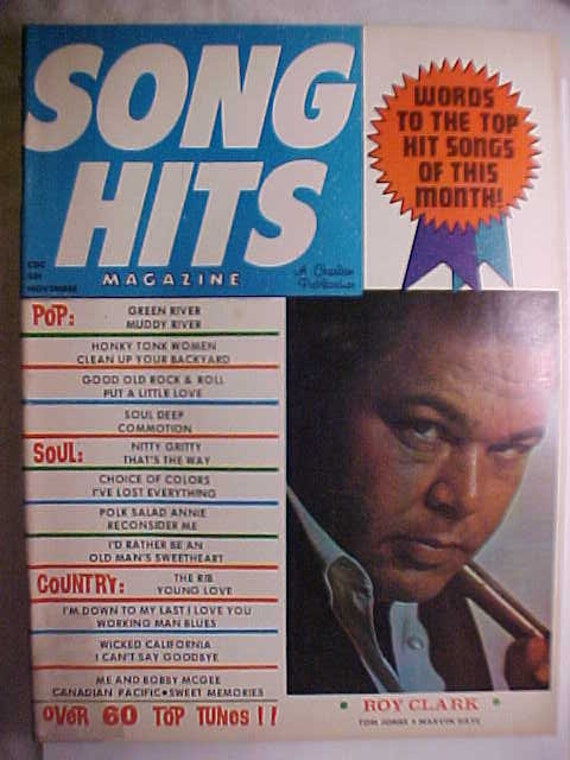This is a vintage magazine cover from the early 1970s. Dominating the top left corner is a large blue square with "SONG HITS" emblazoned in large white letters, and the word "MAGAZINE" in smaller white text beneath it. Adjacent to this blue square on the right is an orange badge featuring a purple and blue ribbon, with the text "WORDS TO THE TOP HIT SONGS OF THIS MONTH" in black at its center. On the left side of the cover, a list of songs spans multiple music genres including pop, soul, and country. These categories are distinguished by their red, funky-looking text. At the bottom of this list, the text "OVER 60 TOP TUNES" also appears in the same red, funky font. The cover features a photo of Roy Clark in the bottom right corner, dressed in a suit and striking a pose with a cane slung over his shoulder. His name is displayed in red text below the photo. The song list includes titles like "Green River," "Funky Young Women," "Doo-Doo-Doo," "Old Rock and Roll," "Soul Beat," "Patty Gritter," "Choice of Colors," "Hulk," "Sal, and Annie," "I'd Rather Be an Old Man," "Sweetheart," "Young Love," "I'm Down to Laugh," "I Love You," "Wicked California," and "Me and Bobby McGee."